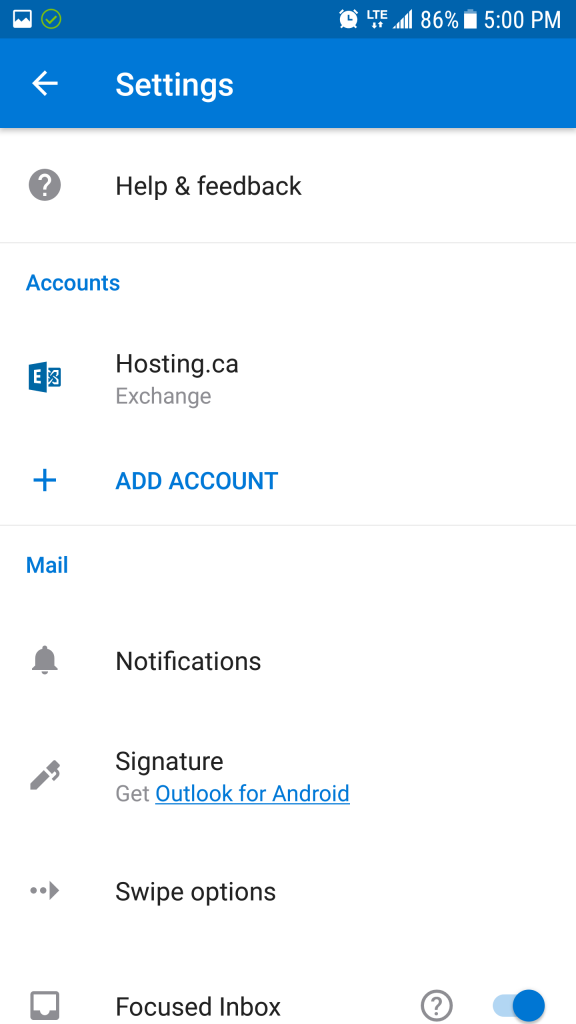In this image, the user is accessing the "Settings" section of an application, which appears to be the Outlook app. The interface shows a predominantly white background with black text, and the top bar is blue, indicating that the user is likely in a mobile version of the app. 

At the top of the settings menu, there are options for "Help and Feedback" followed by "Accounts." The user has an active Microsoft Exchange account listed under a Canadian hosting service (hosting.ca). There is also an "Add Account" button available for the user to include additional email accounts. 

The settings menu continues with a "Mail" subsection that includes various customizable options: 
- "Notifications": Manage how and when email notifications are received.
- "Signature": The current signature is set to "Get Outlook for Android," suggesting that this is the mobile version of Outlook.
- "Swipe Options": Configure swipe gestures for managing emails.
- "Focused Inbox": A toggle switch that is currently activated, meaning the app is prioritizing and displaying emails based on user-defined criteria.

Additionally, there's a back button allowing the user to return to the previous screen. The overall interface design is clean, with intuitive navigation and clarity provided through its text and color scheme.